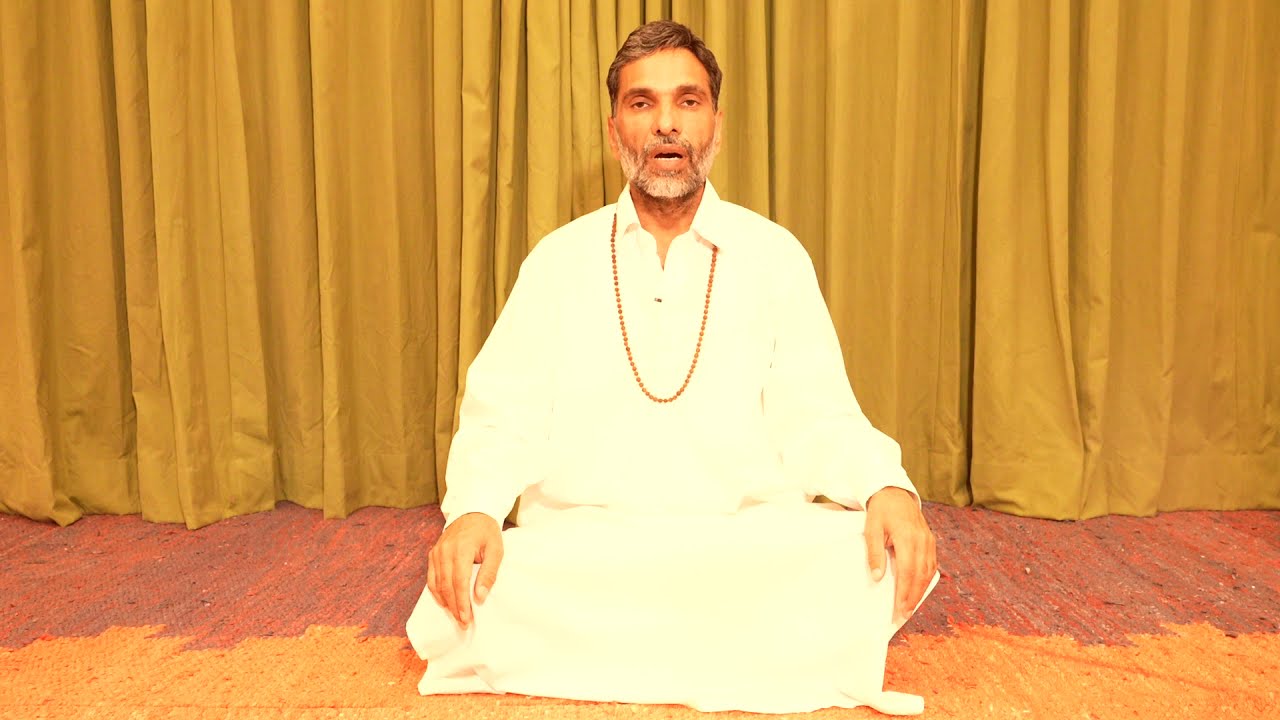This is a horizontally aligned rectangular image of a man, possibly of Indian or Arabic descent, sitting cross-legged on a multicolored floor. He is dressed in a white one-piece outfit with a collar and wears a long gold bead necklace that extends to the middle of his torso. The man appears to be middle-aged, perhaps around 50, with dark hair showing significant graying, and a similarly graying beard. His hands rest on his knees, and he is looking directly at the camera with his mouth slightly open, revealing his bottom teeth. Behind him, there is a tall gold curtain covering the entire background of the image. The floor he is seated on is patterned in patches of reddish-gray and orange with white speckles.